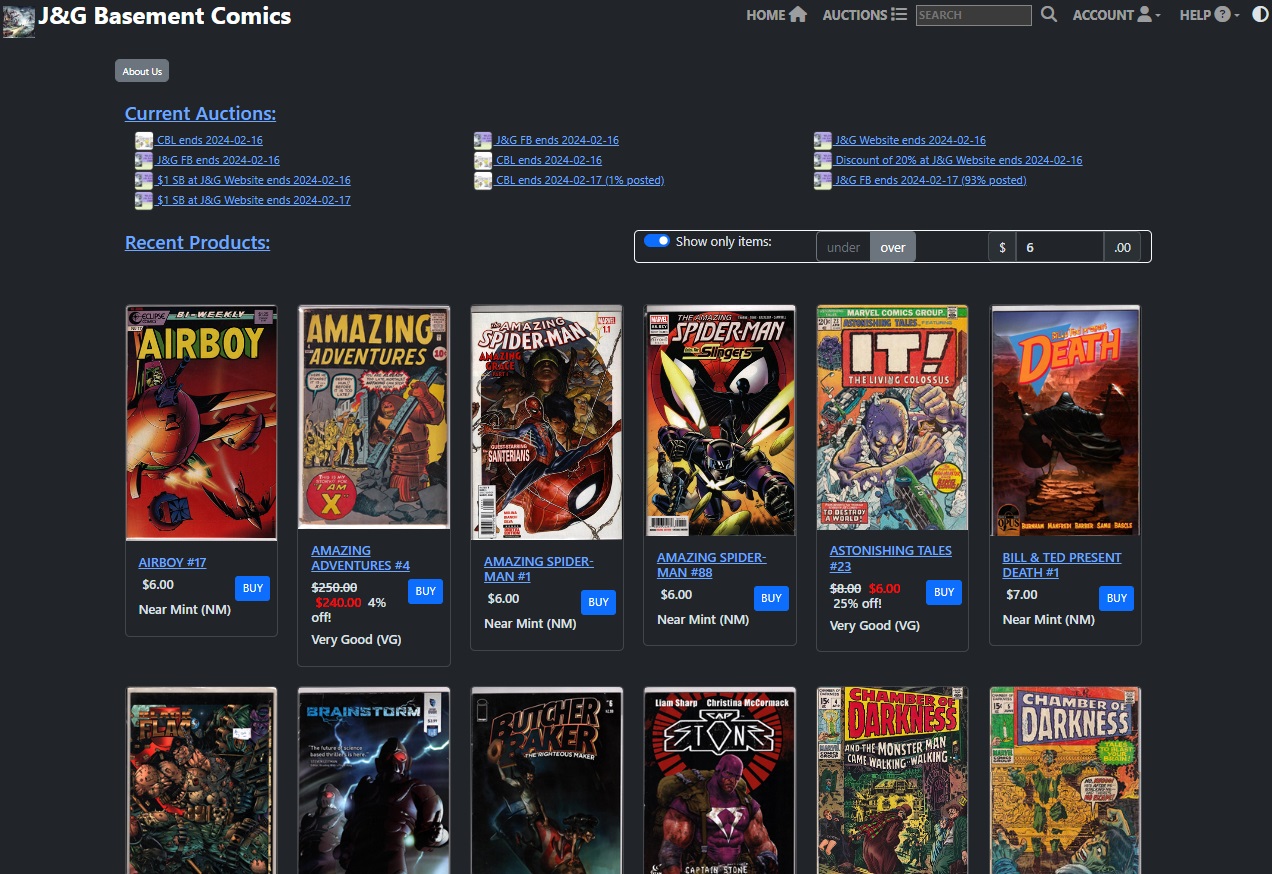The image showcases the webpage of J&G Basement Comics, a specialty comic book store. In the upper left corner, there is a profile picture. To the right, the navigation bar includes links to Home, Auctions, Account, and Help. Just below, there is a gray box labeled "About Us." The background of the website is predominantly black, giving it a sleek look.

The section titled "Current Auctions" displays various comic book icons with descriptive text links in blue, which detail the end times of the auctions. This section is divided into three distinct segments. Beneath this, an option labeled "Show Only Items" is toggled on, and there are additional filters for price ranges "Under" and "Over" with the "Over" option highlighted. A number 5 is entered in this section, accompanied by a $6 filter in the final box.

The area marked "Recent Products" showcases the covers of multiple comics. The first row includes titles like "Airboy," "Amazing Adventures," “Spider-Man,” and “It.” Details such as the pricing of these comics are displayed, with most priced around $6. Notably, one comic originally priced at $250 is marked down to $240. The bottom row also contains comic images, but they are partially cut off.